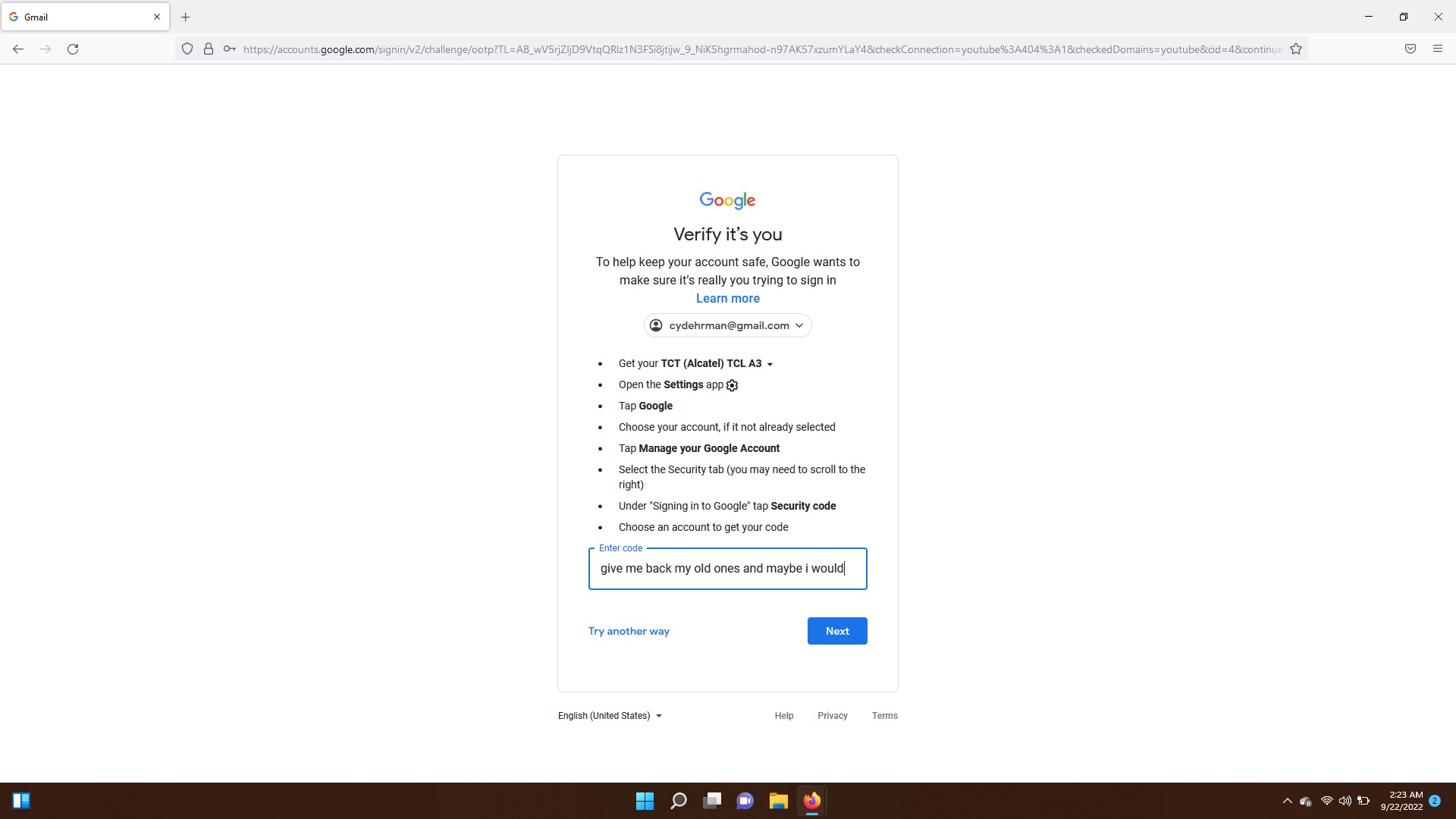The image is a detailed screenshot of a desktop browser displaying a Google account verification page. The webpage, which has a white background, features a large vertical rectangle centrally located on the screen. At the top of this rectangle, the Google logo is prominently displayed. Below the logo, the text "Verify it's you" is visible, followed by a series of bullet points listed vertically down the page. Toward the bottom of the rectangle, there is a text input field labeled "Enter code," accompanied by a blue button with the text "Next." The rest of the webpage is blank, emphasizing the focus on the verification process.

At the bottom of the screenshot, the user's brown taskbar is clearly visible. The taskbar contains icons positioned centrally, including Search, Calculator, Mail, and Firefox. The Firefox icon is highlighted with a blue line underneath, indicating that the Firefox browser is currently open. On the right side of the taskbar, additional system icons such as the Wi-Fi signal, battery status, and the current time and date are displayed. The overall appearance suggests that the user is in the process of verifying their Google account within a Firefox browser window.